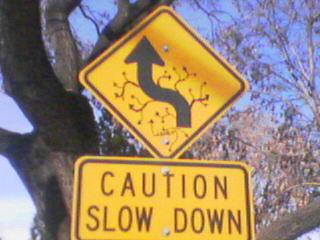The photograph captures a highway sign set against a picturesque backdrop. The central sign features the familiar "S" shaped arrow, indicating an upcoming left and right turn. Below it is a rectangular, yellow caution sign urging drivers to slow down. The upper portion of the image reveals a vibrant blue sky. Dominating the background is a majestic, old-growth oak tree, accompanied by a younger tree, possibly a birch, in the upper right corner. An intriguing modification has been made to the primary sign; someone has meticulously drawn additional branches and smaller arrows onto the main directional arrow, transforming it into a complex flow chart-like illustration. This creative addition of arrows upon arrows extends the original design into an intricate network that almost resembles budding twigs.